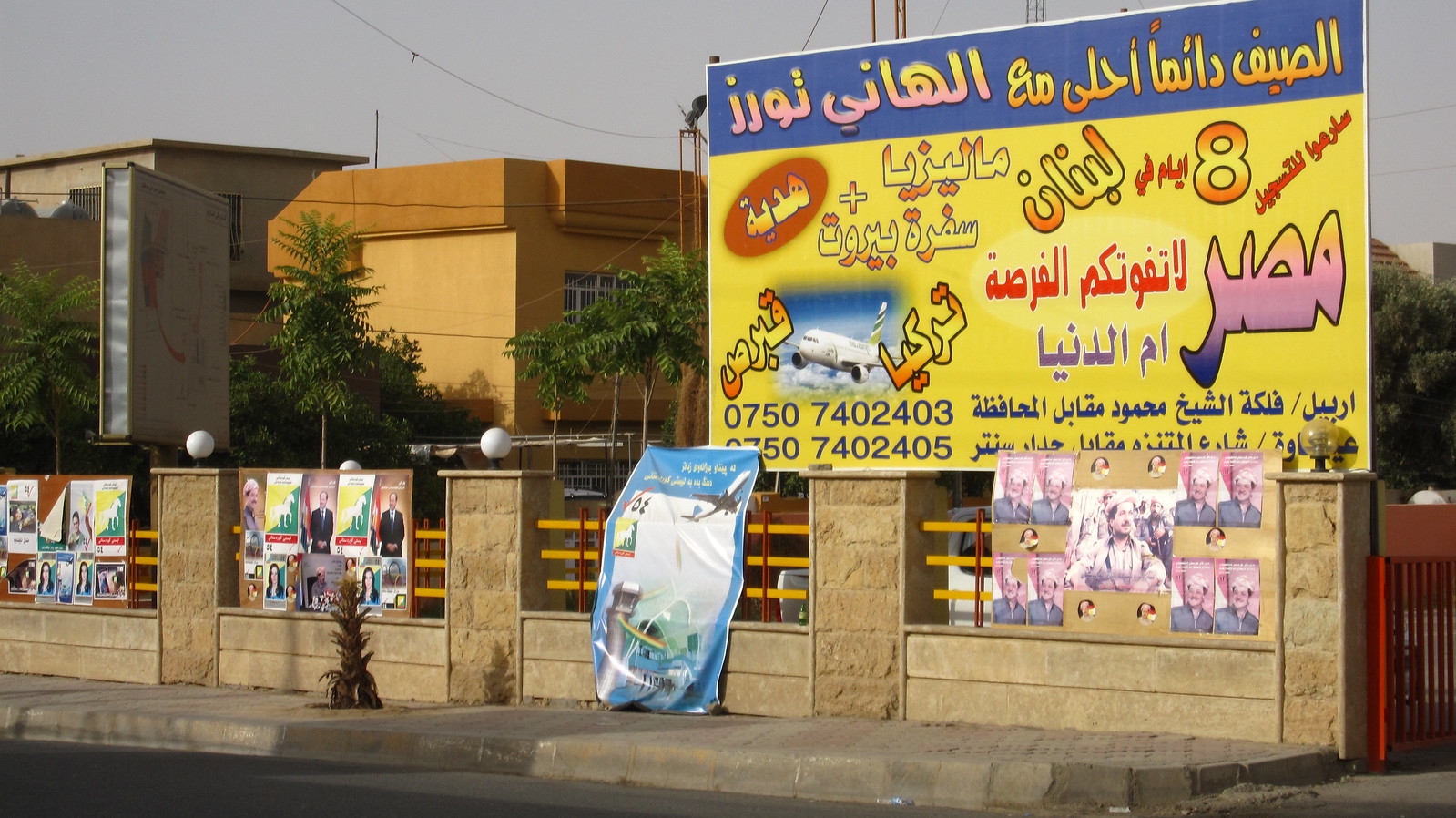This outdoor photograph captures a vibrant city street scene dominated by various advertisements and posters. In the center of the image, towards the bottom, a stone wall with fencing is flanked by stone pillars topped with lights. The fence is adorned with multiple posters, many of which feature a close-up of a man in a suit. To the right, another banner depicts an airport. Above this setup, a large billboard looms, predominantly yellow with blue highlights, containing a mixture of letters and numbers in an Arabic or similar script, and prominently featuring an image of an airplane. Below the billboard, additional posters show a man wearing a head wrap, looking to the left. In the distant background, a mix of trees and buildings, including a distinctive orange and yellow building to the left of the billboard, punctuates the gray sky. The overall scene is rich with urban elements and detailed advertising.